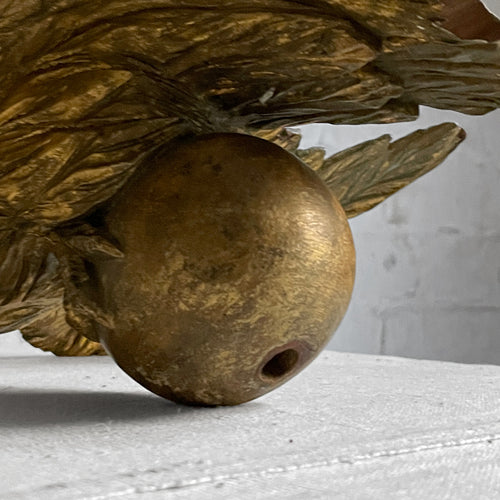The image depicts a detailed sculpture of a bird, likely an eagle, carved from wood but finished with a gold or bronze glaze. The bird's lower section, including its well-defined feathers and menacing claws, is prominently displayed, gripping a large, shiny brass sphere. This sphere, which has varying shades of gold and a slightly scratched surface, features a noticeable circle hole. The sculpture rests on a solid, white-gray stone table. The background consists of a white brick wall, adding to the stark and minimalist setting of the scene. There are no additional elements or lettering in the photograph, allowing the intricate details of the bird's talons, the texture of the feathers, and the gleaming sphere to dominate the composition.